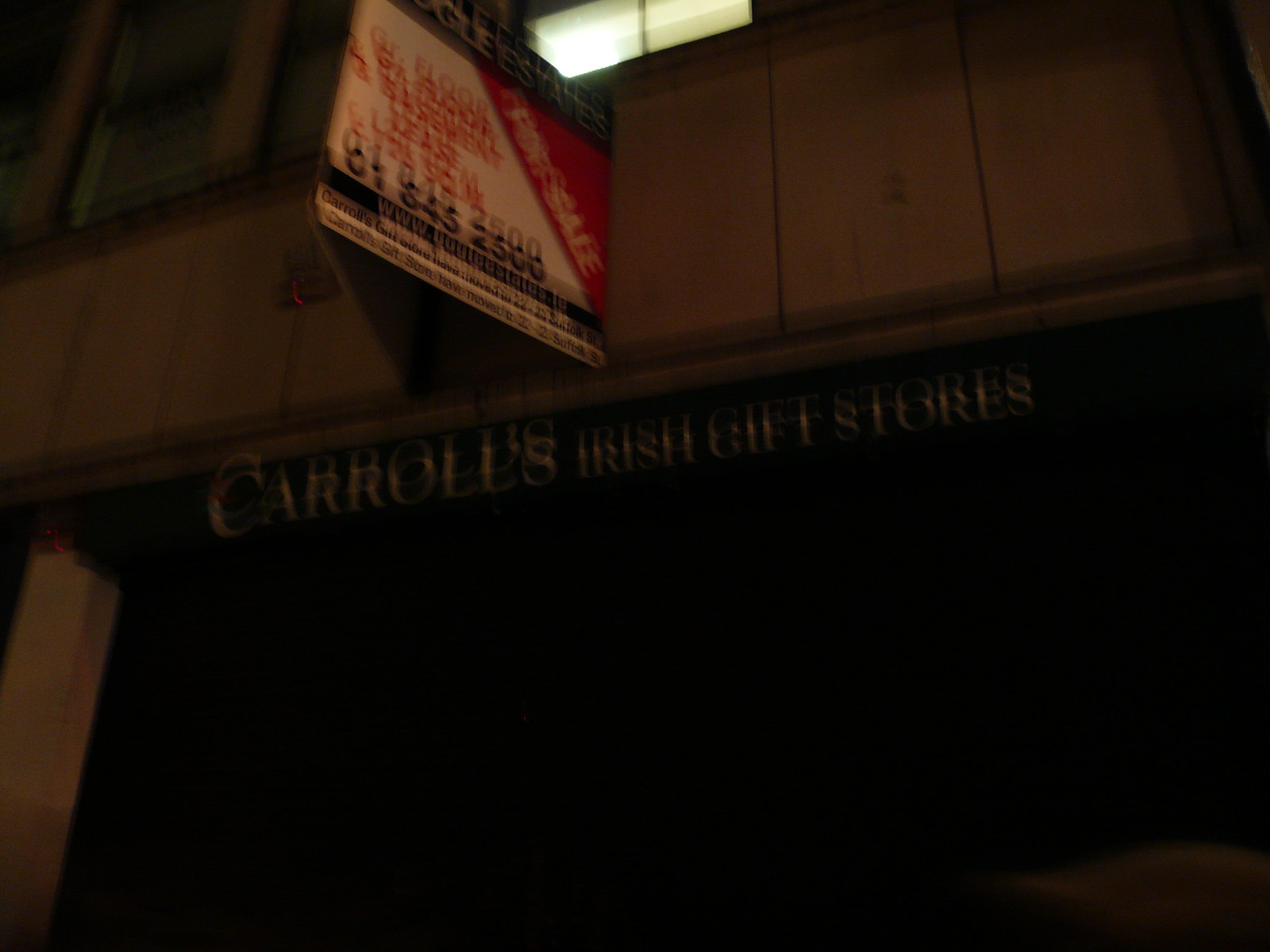A poorly captured nighttime photograph depicts a gray stone building with large rectangular blocks forming its exterior walls. The name "Carroll's Irish Gift Stores" is displayed across the top, although the text is very blurry and distorted due to camera movement. Below the signage, a black gate can be seen at the base of the building. Above the store's name, there's a protruding sign shaped like two extending triangles, which contains a phone number and additional, illegible text. A single white light shines from a window at the top of the image, adding a faint glow to the dark surroundings.